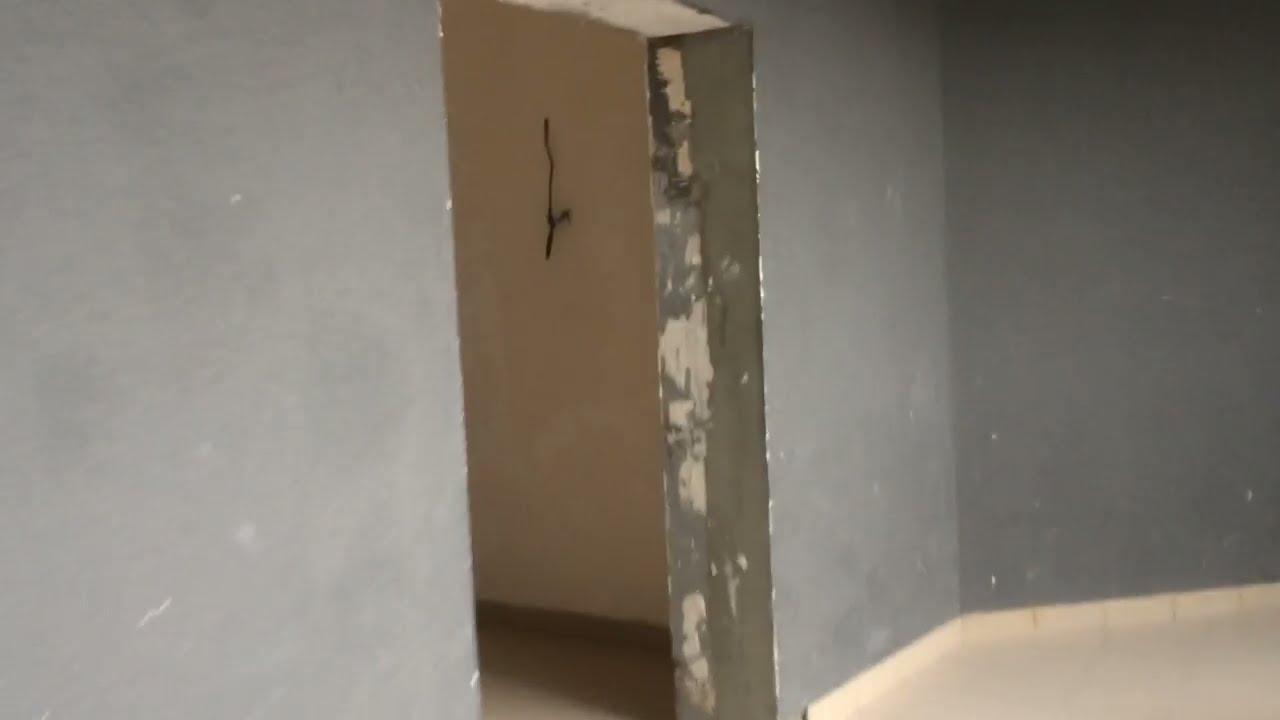The photograph captures a stairwell within a building or apartment complex, showcasing an indoor setting with distinct architectural features. The walls on the left side are white, constructed from a stucco material, contrasting with the brown or beige tiled stairs. The metal railings, composed of three thin, elongated pieces of wire-like metal, provide support on the right. The camera angle is slightly tilted, offering a unique perspective as the viewer looks up the staircase from approximately three steps below a flat walkway. This walkway leads to an open, doorless exit or balcony area bordered by a black wire fence. Sunlight fills the space, streaming in from the opening at the top of the stairs, and illuminates the scene with natural light. Outside, glimpses of green tree leaves add a hint of nature to the otherwise structured environment, emphasizing the connection between indoor and outdoor spaces.